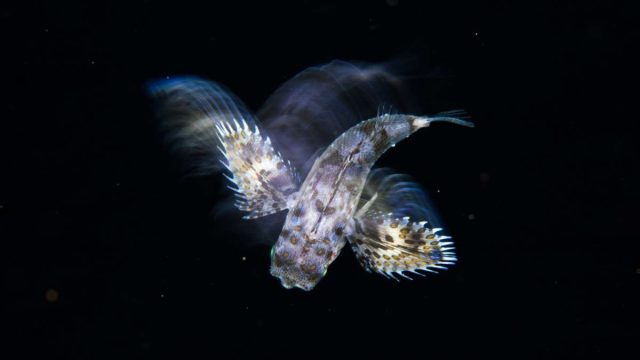This image captures a mysterious sea creature, seemingly deep underwater against an entirely black background. The central focus is a translucent fish with a body predominantly white and blue, exhibiting streaks of both light and dark purple, along with a couple of black dots near its middle. The fish appears to be in motion, evidenced by fluid lines and streaks trailing around its form, giving a dynamic sense of movement. It has a distinctly shaped squared-off upper face with a slight indentation resembling a nose, which transitions into a rectangular midsection and tapers into a pointy tail highlighted with white at the tip. Angular fins extend from each side of the body, edged with small sharp protrusions that likely aid in its propulsion through the water. The creature's head is directed downwards, and the tail points towards the right, with a shadowy appearance behind it, suggesting rapid motion through the depths. The overall image, with its high-definition dimensions, emphasizes the enigmatic and shadowy presence of this deep-sea fish against the stark contrast of the dark ocean.